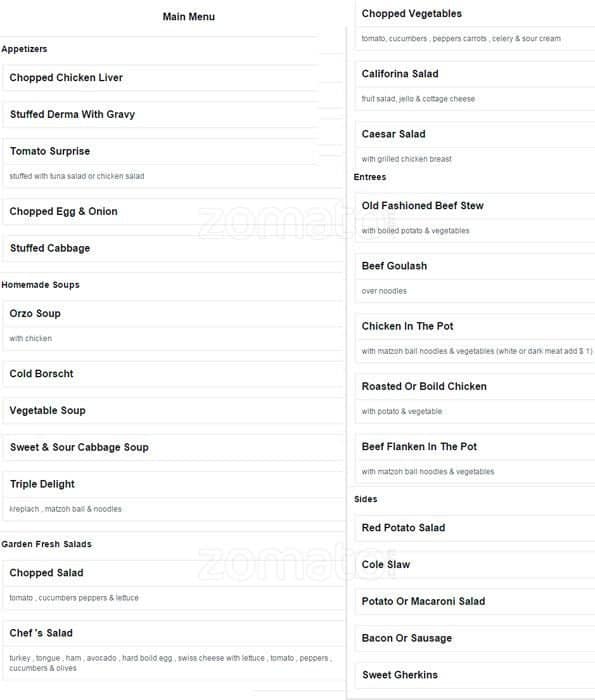This is a detailed description of a restaurant menu. The background is a clean white, and the text is uniformly black. Dish names are highlighted in bold, while their descriptions are in a slightly smaller, non-bold font. The menu is organized into two columns, beginning at the top left corner and running down to the bottom before starting anew at the top of the right column.

At the top center of the menu, "Main Menu" is prominently displayed. Just below it, on the far left, is the section titled "Appetizers." This section features:

- Chopped Chicken Liver
- Stuffed Derma with Gravy
- Tomato Surprise (described as stuffed with tuna salad or chicken salad)
- Chopped Egg and Onion
- Stuffed Cabbage

Following the appetizers is the "Homemade Soups" section, which includes:

- Orzo Soup with Chicken
- Borscht
- Vegetable Soup
- Sweet and Sour Cabbage Soup
- Triple Delight (described as kreplach, matzo ball, and noodles)

Continuing down, the "Garden Fresh Salads" section offers:

- Chopped Salad (tomatoes, cucumbers, peppers, and lettuce)
- Chef Salad (turkey, tongue, ham, avocado, hard-boiled eggs with cheese, lettuce, tomatoes, peppers, cucumbers, and olives)

Beginning at the top of the right column, the menu lists:

- Chopped Vegetables (tomatoes, cucumbers, peppers, carrots, celery, sour cream)
- California Salad
- Fruit Salad
- Jello and Cottage Cheese
- Caesar Salad with Grilled Chicken Breast

For entrees, the options are:

- Old-Fashioned Beef Stew (served with boiled potato and vegetables)
- Beef Goulash (over noodles)
- Chicken in the Pot (with matzo ball, noodles, vegetables; white and dark meat available for an additional $1)
- Roasted or Boiled Chicken (with potato and vegetable)
- Beef Flanken in the Pot (with matzo ball, noodles, and vegetables)

The menu also includes a variety of sides:

- Red Potato Salad
- Coleslaw
- Potato or Macaroni Salad
- Bacon or Sausage
- Sweet Gherkins